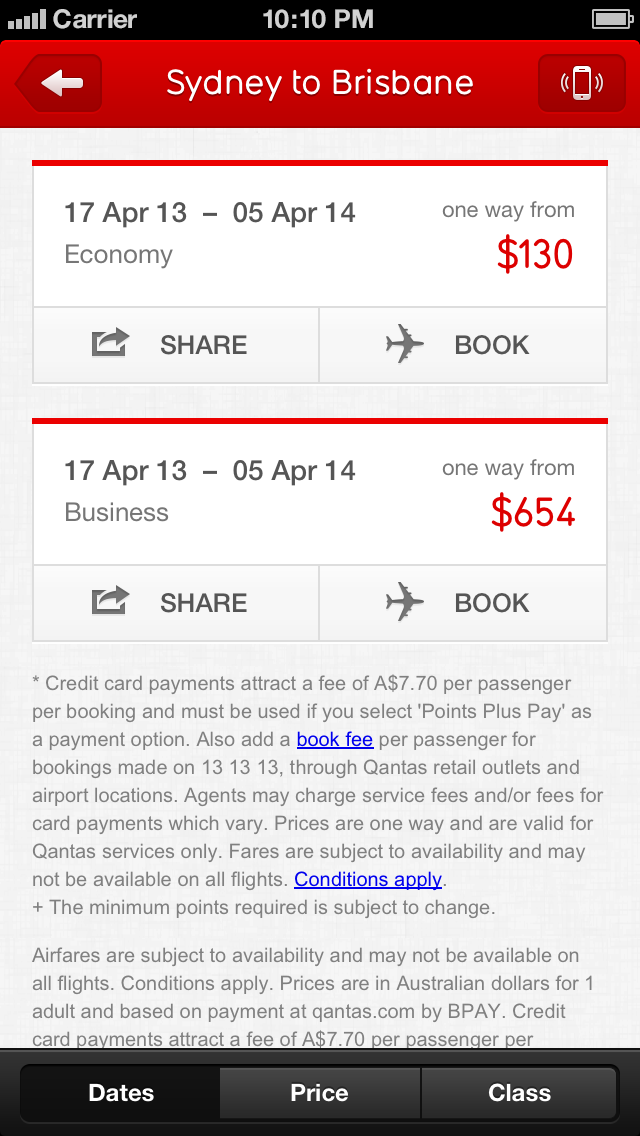A detailed caption for the described image could be:

---

The image features a smartphone screen displaying a flight search result for travel from Sydney to Brisbane. At the top, the status bar shows full signal strength with five bars, the time as 10:10 PM, "Carrier" beside the signal indicator, and a fully charged battery icon on the far right.

Below the status bar, the screen shows a search result header with "Sydney to Brisbane" and a back arrow icon on the left to return to the previous page. To the right of the header, there is an icon depicting a vibrating phone, possibly indicating an active alert.

The first flight option listed is an economy one-way ticket priced from $130, with travel dates from April 13th to April 14th, 2017. Options to share this flight detail and to book the flight are located underneath, with corresponding icons—a share symbol and an airplane icon labeled "Book."

The second flight option shows a business class one-way ticket priced at $654, also with travel dates from April 13th to April 14th, 2017. As with the first, there are options to share and book this flight displayed.

At the bottom of the screen, fine print includes an asterisk explaining credit card information, extra booking fees, conditions, minimum points required, and notes on availability. Additional options to view more flight details by filtering dates, prices, and class are also available at the bottom of the screen.

---